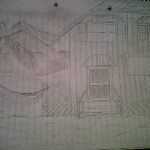This finely detailed pencil drawing depicts a quaint two-story house with a lightly colored facade, nestled amidst a serene landscape with distant mountains silhouetted in the background. The house features a single window on the second floor, providing a glimpse into its upper level. Leading up to the front entrance are a couple of modest steps. The foreground is sparingly populated with what appears to be grass, hinting at a tranquil, rural setting. The artwork is rendered on a grayish beige paper, lending an antique, textured quality to the piece. The artist's mastery in using various shades of pencil brings depth and dimension to the drawing, suggesting subtle coloring without overpowering the natural hues of the paper.